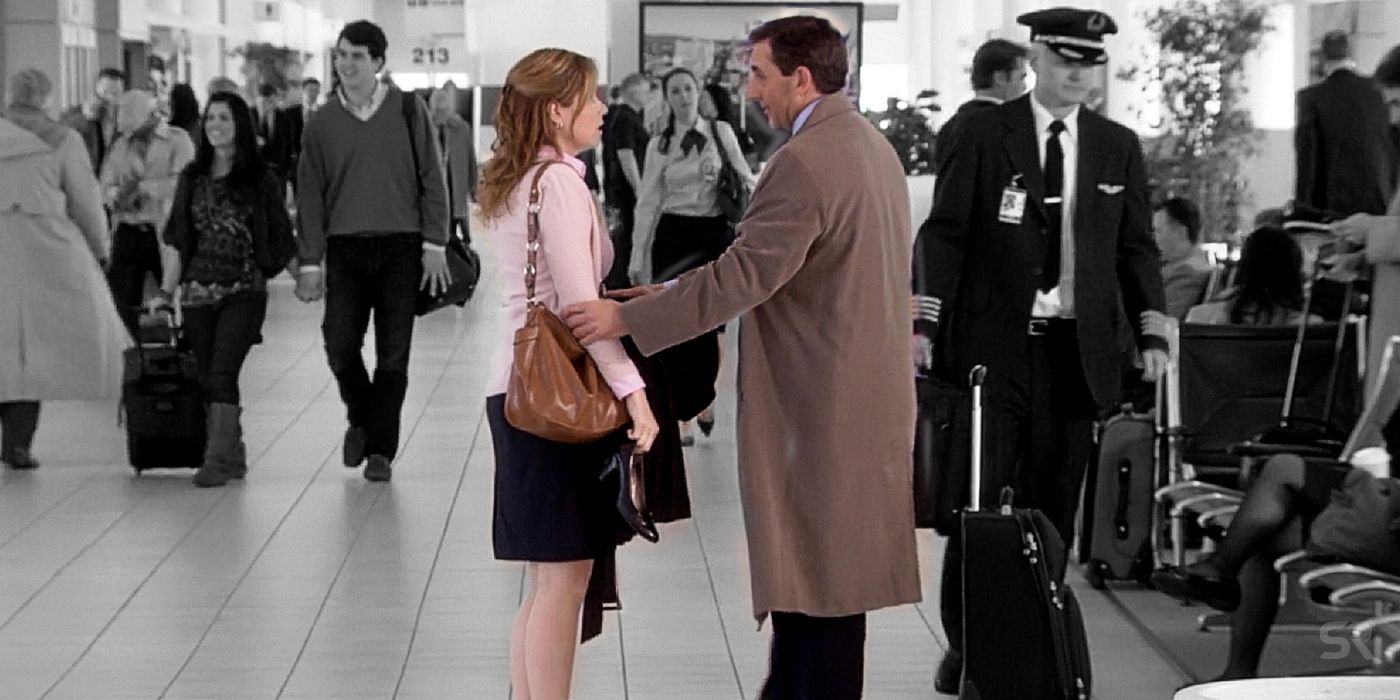In this detailed black and white photograph taken in an airport, we see a bustling corridor lined with travelers carrying bags and luggage, with a sign reading "213" visible above a door at the back. Amongst the grayscale crowd, two individuals stand out vividly in color at the center of the image, bringing immediate attention to their interaction. The man, who bears a resemblance to Steve Carell's character from "The Office," is clad in a long, light brown trench coat and black pants. He is reaching out to hold the arms of a woman, who appears to be Pam from the same show. She has light brown, long wavy hair pulled back with a clip, and is wearing a pink blouse, a black skirt, and a light brown leather purse over her shoulder. Her expression is one of surprise or upset as she looks at him.

In the background, detailed elements include a man in a uniform with a military pin and a hat walking on the right side, and various other travelers engaged in typical airport activities, such as holding hands, dragging luggage, and seeking assistance from personnel. Additionally, there is an airline captain walking towards the camera and seating areas to the right side of the image. Despite the surrounding commotion of travelers all represented in black and white, the intimate and colored scene between the man and woman at the center captures a poignant and cinematic moment within the everyday hustle of an airport.